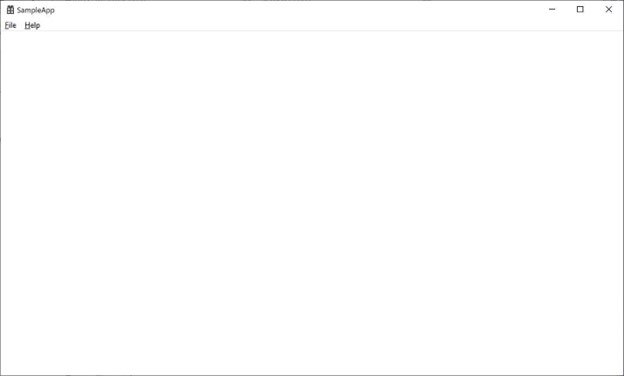This image depicts a rectangular interface in landscape orientation, bordered by a thin black outline. Positioned approximately half an inch from the top is a slim, light gray horizontal line extending across the entirety of the rectangle. In the upper left corner, there is a small gift icon next to the text "SAMPLE APP," with both words fully capitalized. Directly below this, two menu headers labeled "File" and "Help" appear, each word capitalized with an underscore beneath the initial letter. In the upper right corner of the rectangle, there are four small symbols: a hash (#), a dash (-), a small square (□), and a small ‘x’ (×).